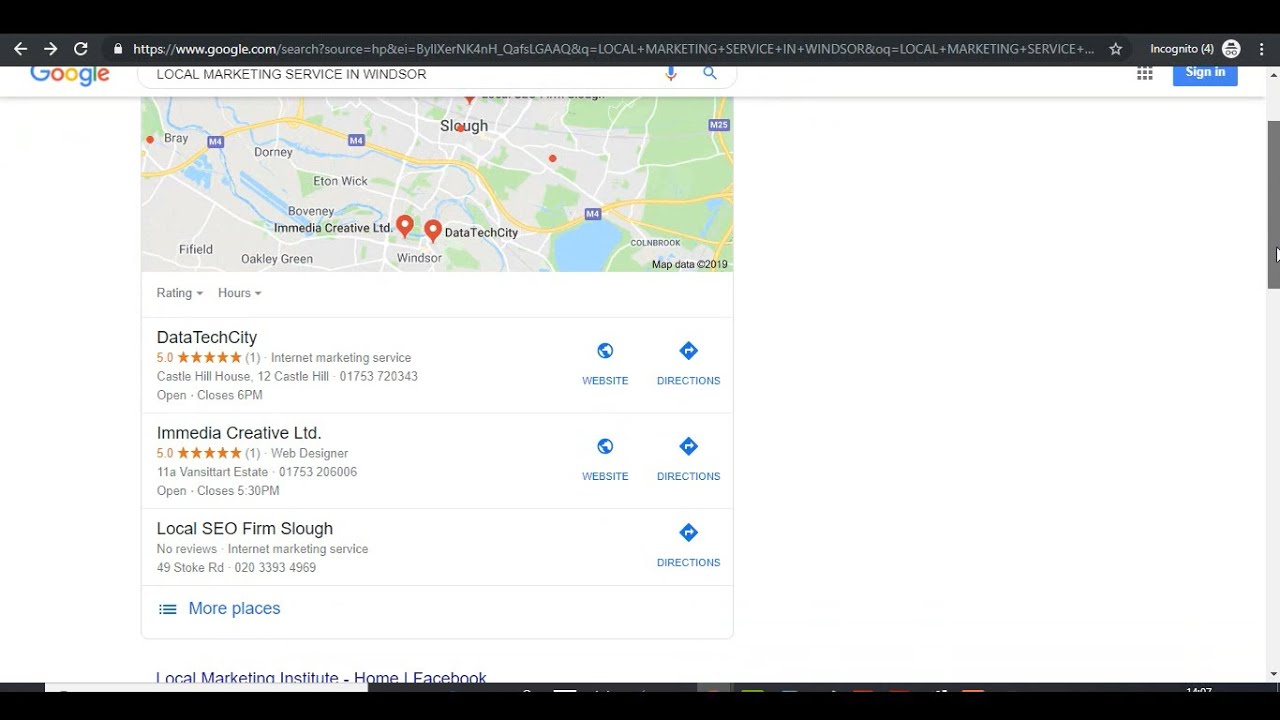A detailed and cleaned-up descriptive caption for the provided image could be:

"This screenshot from google.com captures a search for local marketing services in Windsor. In the browser's top search bar, the query 'local marketing service in Windsor' is visible. Below, a map is displayed with red markers indicating the locations of the top three search results.

The first result is 'Data Tech City,' identified as an internet marketing service. It features a review, the company's address, phone number, operational hours, and blue links for both their website and directions.

The second result, 'Emedia Creative LTD,' is listed as a web designer. This entry includes a review, along with the company's address, phone number, hours of operation, and blue links to their website and directions.

The third result is 'Local SEO Firm Slow,' categorized as an internet marketing service. Unlike the others, it has no reviews and only provides the address and phone number, with a blue link available for directions but none for a website."